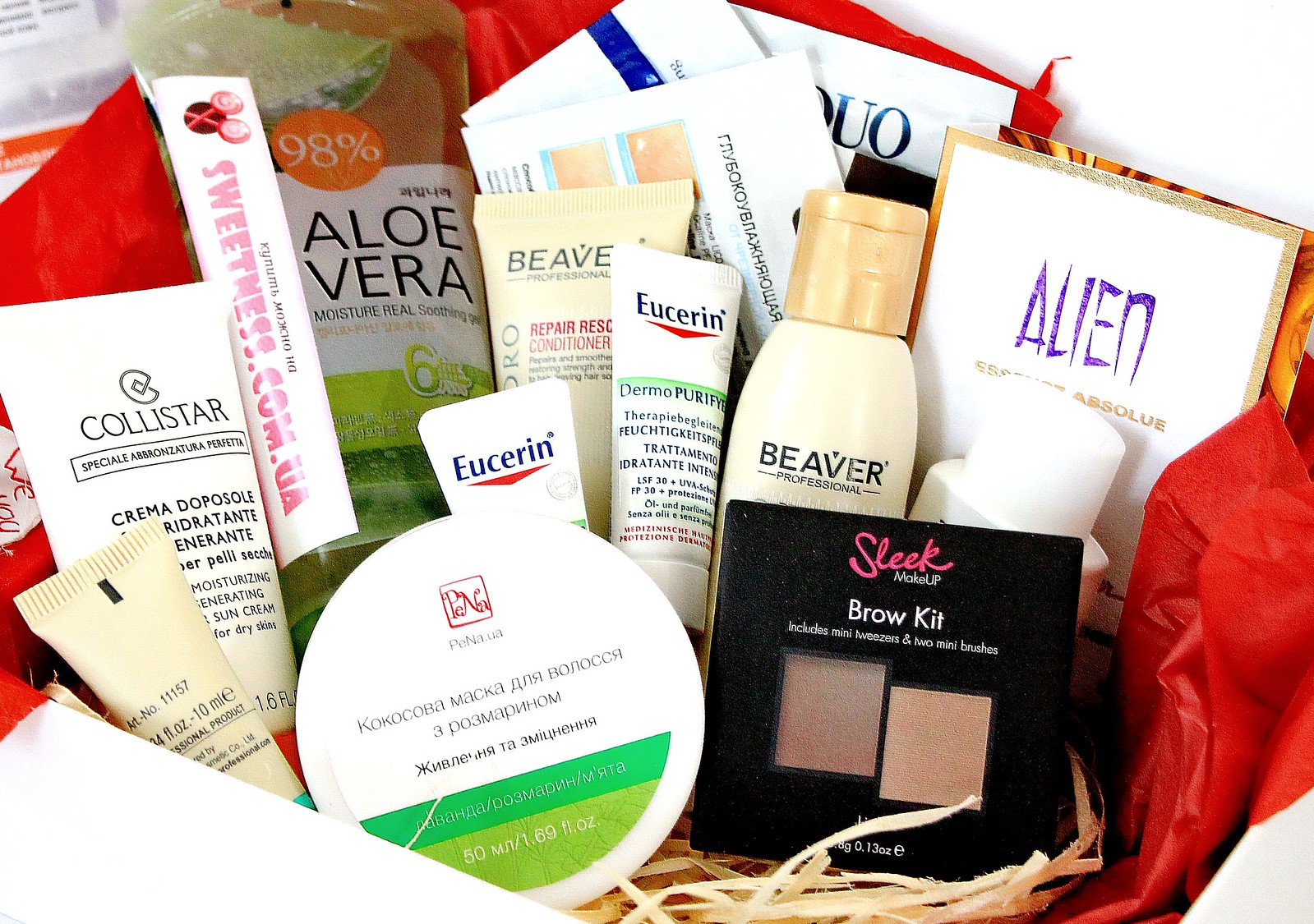In this detailed photograph, we observe an intricately assembled gift basket, thoughtfully lined with straw at the bottom and accented with vibrant red tissue paper. This basket is brimming with an assortment of skincare products neatly arranged for display. Prominently positioned at the back is a tube labeled "Aloe Vera," designed with clean, white packaging accentuated by green stripes. In the foreground, there are two smaller tubes clearly marked with "Eucerin," featuring a distinctive red triangle and the label "Dermal Purify," accompanied by additional descriptive text. Near the bottom of the basket lies a round container, roughly the size of a shoe polish kit, with a white exterior and an array of Cyrillic script on it. This container also displays green stripes and the measurement of 50 ml (1.69 fluid ounces). Adjacent to it, on the right, is a sleek, black square box identified as a "Sleek Makeup Brow Kit," which includes mini tweezers and two mini brushes. This careful arrangement of diverse skincare items within a delicately crafted gift basket exemplifies a perfect gift for skincare enthusiasts.